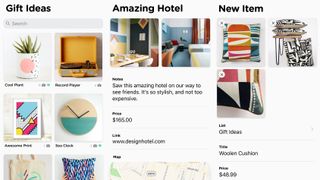The image depicts an online store layout divided into three sections. The left section, titled "Gift Ideas," features six products, although only the top four are fully visible. Under this heading:

1. A white and pink ceramic cup or pot plant containing a green plant.
2. An orange suitcase.
3. A white page decorated with drawings in blue, red, and yellow, with accents of red and grey.
4. A world clock with a brown upper half and a blue bottom half, featuring black clock hands.

The remaining two products under "Gift Ideas" are partially obscured and not fully visible.

The middle section, labeled "Amazing Hotel," showcases images of hotel room decorations with a listed price of $65. However, the text and description are blurry and not easily readable.

The right section, titled "New Items," features black and white pillows priced at $46.99.